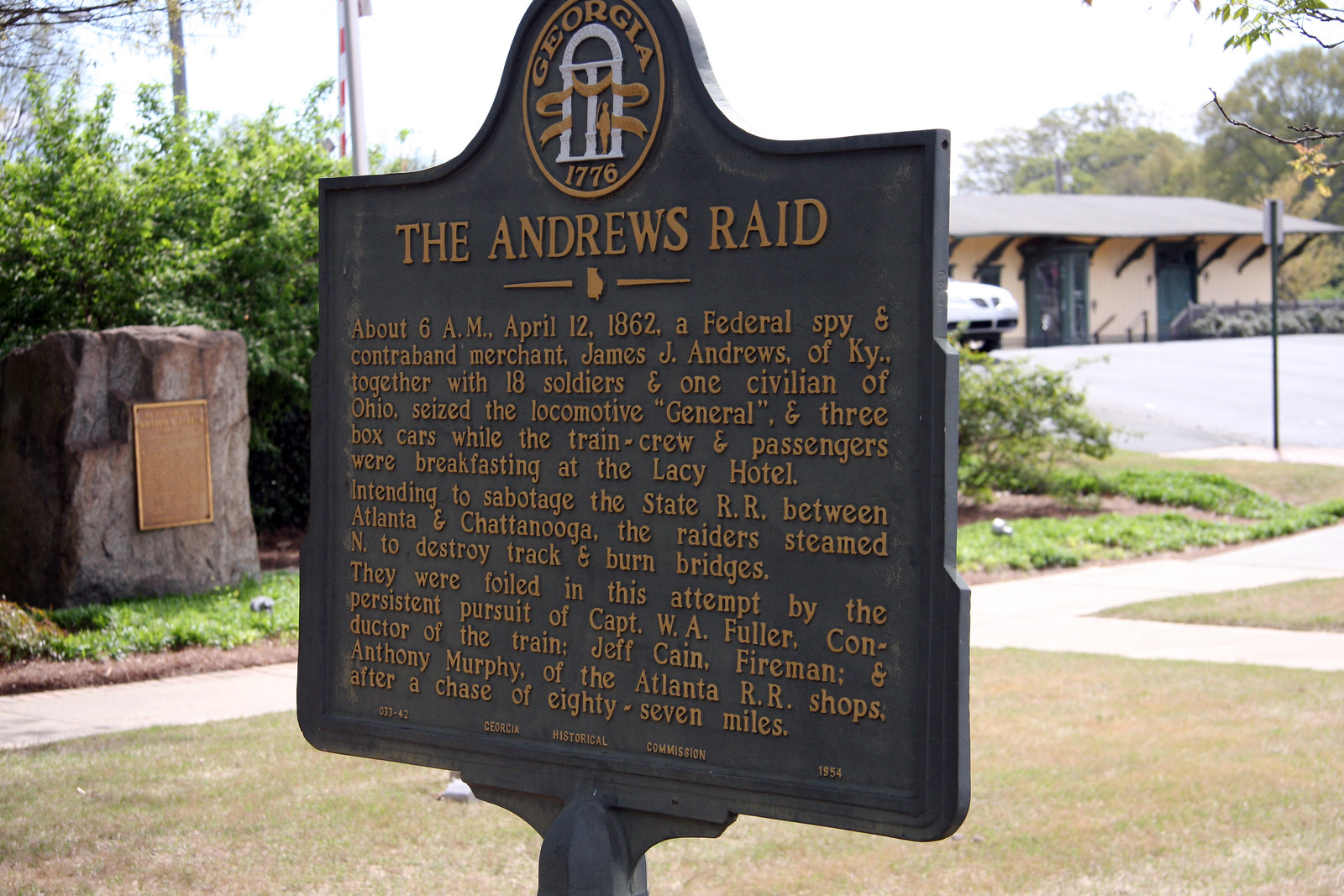This horizontal, rectangular photograph centers on a large historical marker set in a neighborhood, possibly a park. The marker is dark blue with gold writing. Prominently at the top, the text reads "Georgia, 1776" and "The Andrews Raid." Above this, there is a circular emblem, likely representing the society that placed the marker. Surrounding the marker is a scene of green grass and trees, with a house and driveway visible on the right, suggesting a residential or business area. A silver car is parked in the background.

The text on the marker provides a detailed account of an event known as the Andrews Raid. It recounts how on April 12, 1862, at approximately 6 a.m., James J. Andrews, a federal spy and contraband merchant from Kentucky, along with 18 soldiers and one civilian from Ohio, seized the locomotive General and three boxcars while the train crew and passengers were breakfasting at the Lacey Hotel. Their intent was to sabotage the state railroad between Atlanta and Chattanooga by destroying the tracks and burning bridges. However, their mission was thwarted by the persistent pursuit of Captain W.A. Fuller, the train's conductor, Jeff Kane, the fireman, and Anthony Murphy of the Atlanta Railroad shops, ending in a chase that spanned 87 miles.

In the background, across the road, there is another historical marker mounted on a boulder, also featuring a plaque, adding to the historical ambiance of the setting.